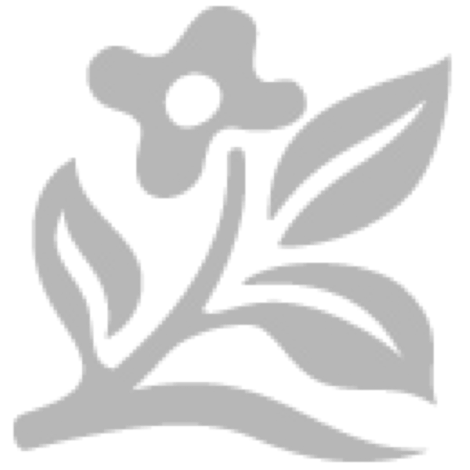This close-up photo, taken during the day in a large garden area, features a vivid field of unique magenta-pink flowers that stand out dramatically against the surrounding greenery. The flowers, resembling miniature trees with their long stems crowned by conical clusters of tiny blossoms, rise amidst a sea of dark, pointy leaves tinged with a bluish hue. These striking, bright pink flowers create a stunning contrast against the tall green grass and diverse bushes in the background. The perspective appears to be a bird's-eye view, highlighting the dense patch of these intriguing flowers, which are both unfamiliar and captivating, possibly prompting the photographer to capture their beauty and uniqueness.